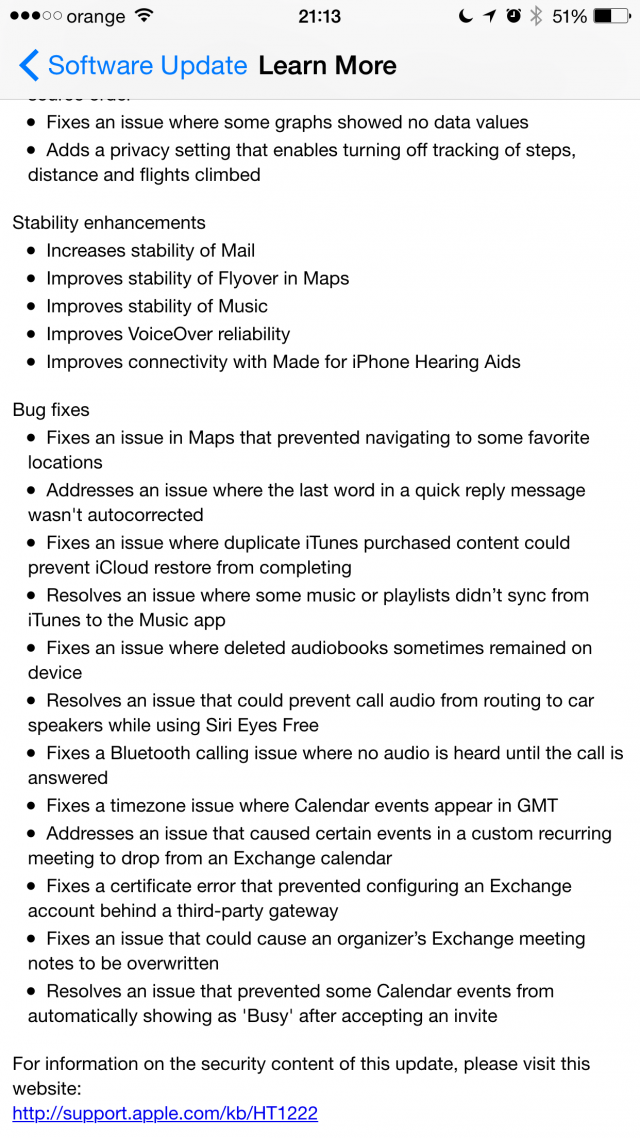**Detailed Caption:**

This is a screenshot of a smartphone screen that features an update notification. The top of the screen has five status icons arranged from left to right: three black icons (a Wi-Fi signal, a timestamp showing 21:13, and a moon icon), followed by a black send icon, a black clock icon, a grey Bluetooth icon, and a battery icon indicating 51%.

Below the status bar, a blue bar contains a left-facing arrow, the text "Software Update" in blue, and a "Learn More" link to the right. 

The main content is a detailed list of updates and improvements provided in bullet points, including:
- Fixes an issue where some graphs showed no data values.
- Adds a privacy setting for turning off tracking of steps and distance.
- Stability enhancements.
- Increases stability of Mail.
- Improves stability of Maps.
- Improves stability of Music.
- Improves VoiceOver reliability.
- Improves connectivity with Made for iPhone hearing aids.
- General bug fixes including:
  - Fixes an issue in Maps preventing navigation to some favorite locations.
  - Addresses an issue where the last word in quick replies was not auto-corrected.
  - Fixes an issue preventing iCloud restore due to duplicated iTunes-purchased content.
  - Resolves an issue where music/playlists did not sync from iTunes to the Music app.
  - Fixes an issue where deleted audiobooks sometimes remained on the device.
  - Resolves an issue preventing call audio from routing to car speakers while using Siri Eyes Free.
  - Fixes a Bluetooth calling issue where no audio was heard until the call was answered.
  - Addresses a time zone issue with calendar events appearing in GMT.
  - Addresses an issue causing certain events in a custom recurring meeting to drop from an Exchange calendar.
  - Fixes a certificate error preventing configuring an Exchange account behind a third-party gateway.
  - Fixes an issue that could cause an organization's Exchange meeting notes to be overwritten.
  - Resolves an issue preventing some calendar events from automatically showing as "busy" after accepting.

For more information or the security content of this update, a link to support.apple.com is provided.